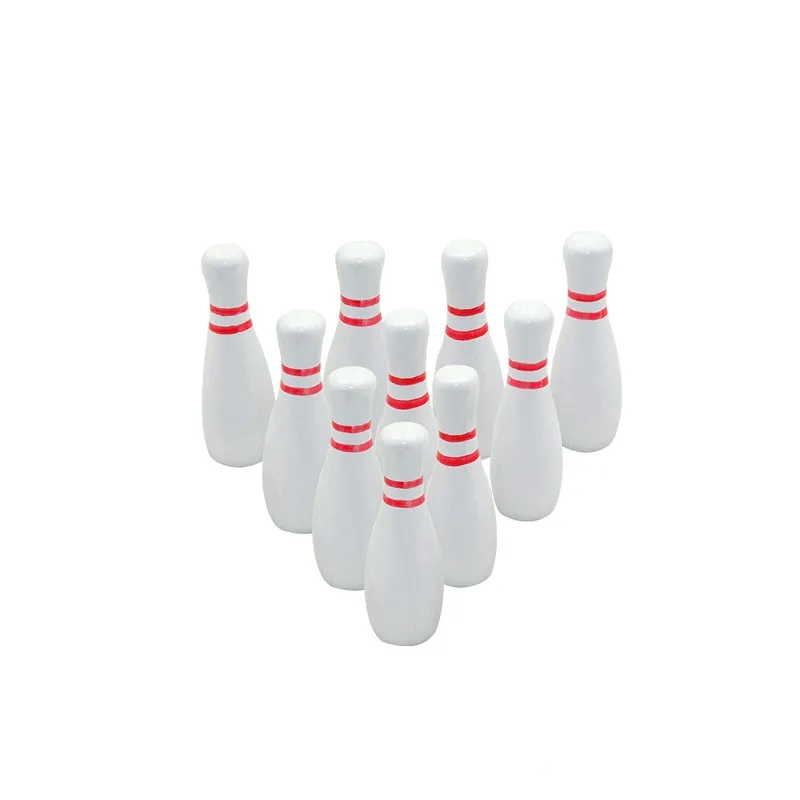The image depicts a set of ten bowling pins arranged in a traditional triangular formation on a plain white background, akin to a bowling alley setup. Each pin is colored white and features two red stripes encircling the neck, characteristic of standard bowling pins, but they exhibit slight wear, with some white showing through the stripes. The pins are organized with one pin at the front, followed by rows of two, three, and four pins respectively. The setting suggests a simplistic, almost graphic art or clip art style, with a slight glare at the top of the pins making them appear a bit shorter than usual. There are no additional elements or text present in the image, emphasizing the pins themselves as the sole focus.